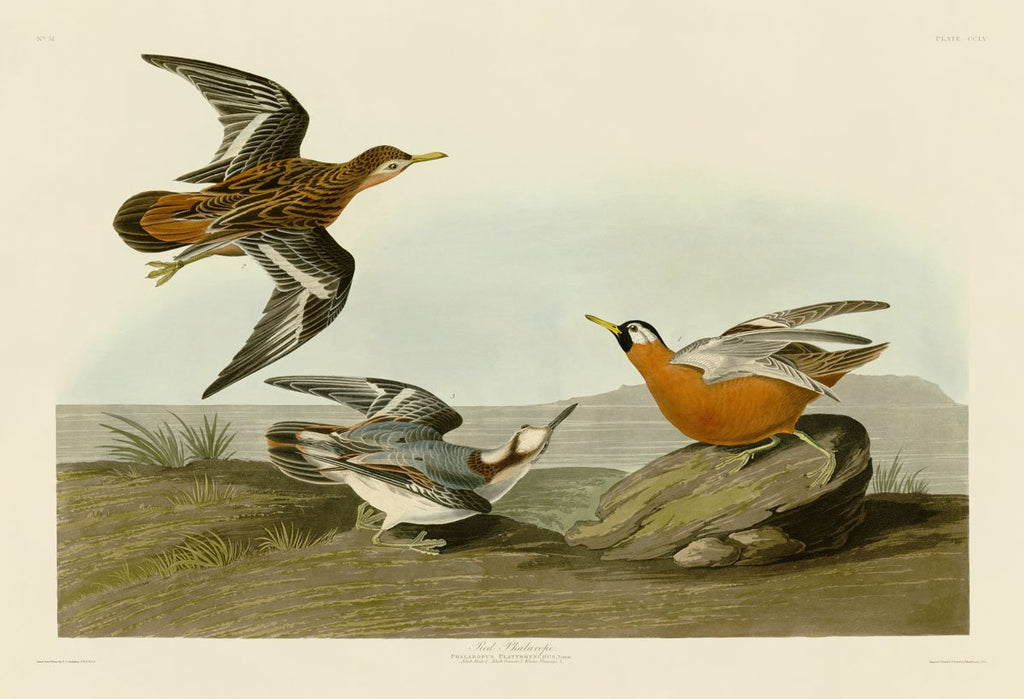This image is a traditional-style painting featuring three distinct birds set against a tan and subtly greenish-blue sky. The artwork appears to draw on old Japanese painting techniques, with notable text and markings presumably indicating the painting and artist's name in various handwritten fonts on the borders.

The scene is set on a tan to grayish, slightly grassy ground, possibly depicting a mountainous or cliffside environment. The focal points of the painting are the three birds, each carefully detailed to convey uniqueness.

One bird is airborne in the upper left corner, characterized by its brown body with a yellow beak. Its wings are black adorned with white patterns.

On the ground to the left center, there is a cream-colored bird with a gray-blue and brown hue. Its head is white, and it has a darker beak, with a white underbelly and gray on top.

The third bird perches on a moss-covered rock in the bottom right. This bird features a yellow beak, black head with white around its eyes, and a light brown body with gray, cream, and brown wings.

The backdrop of the sky is primarily tan, transitioning into shades of greenish-blue and gray, evoking an overcast ambiance. Small, short grassy areas and bits of plant life enhance the rugged, natural setting.